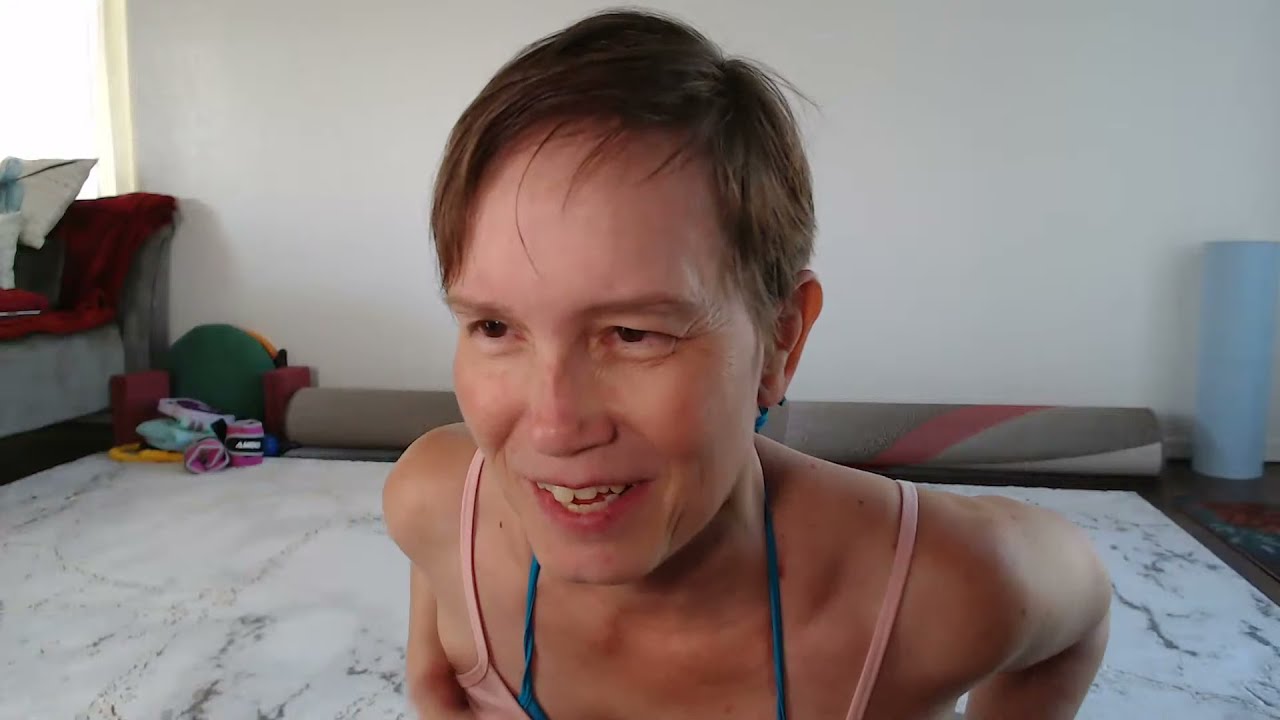A Caucasian woman with short brown hair, parted on the right and combed over to the left, is sitting at the edge of a bed with a solemn expression. She is wearing a pink tank top over a teal one, the straps of both visible on her pale shoulders. She has brown eyes, and her mouth is open, revealing her teeth, one noticeably longer than the other. The background features a mixture of home furnishing elements: a white wall with no decorations, rolled-up carpets of various colors and designs, and a gray couch partially covered with a red throw and several pillows. A window on the left allows light to stream into the room, illuminating a pile of indistinct cloth objects beneath it and adding a splash of natural brightness to the otherwise stark setting. The floor beneath her appears to have a marble-like texture, white with black swirls, contributing to the clean and minimalist appearance of the space.